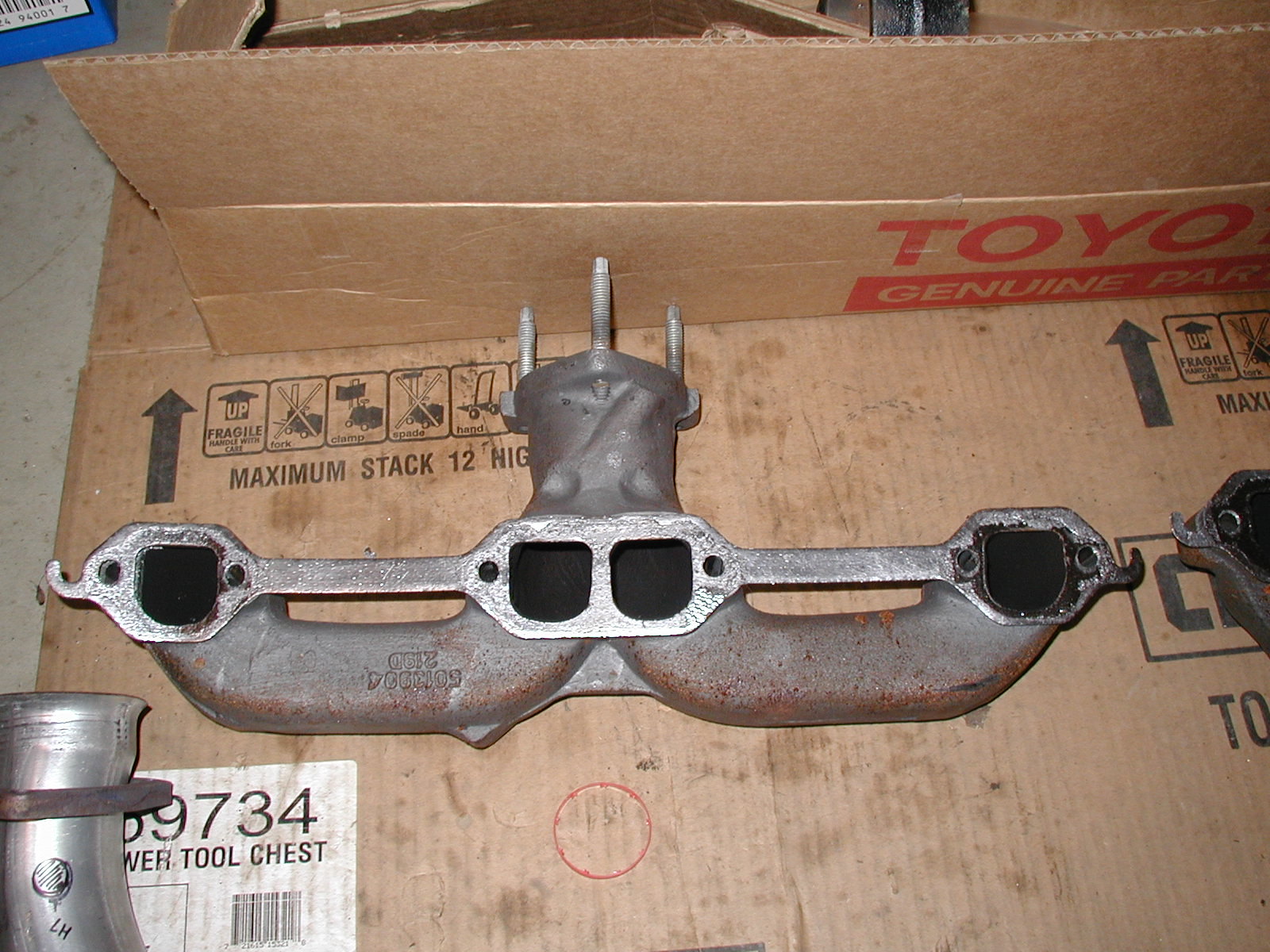This color photograph depicts a dirty metal car part, reminiscent of a vehicle component potentially meant for a Toyota, as suggested by the red "Toyota Genuine Parts" text on the worn cardboard box it rests upon. The gray metal assembly resembles a large, fragmented W, with multiple sections diverging into various openings — four large blackened openings, two central openings, and other smaller ones. The part is secured with three prominent screws at the bottom, indicating it might be a fixable or replaceable component. In the cluttered scene, additional metal parts are noticeable to the right and bottom left, accompanied by a white tag with the number 9734 and the word "tool chest." The cardboard box dominates the horizontal frame, marked with usage warnings and stacking instructions beneath the metal piece, all placed on a dirty concrete surface.